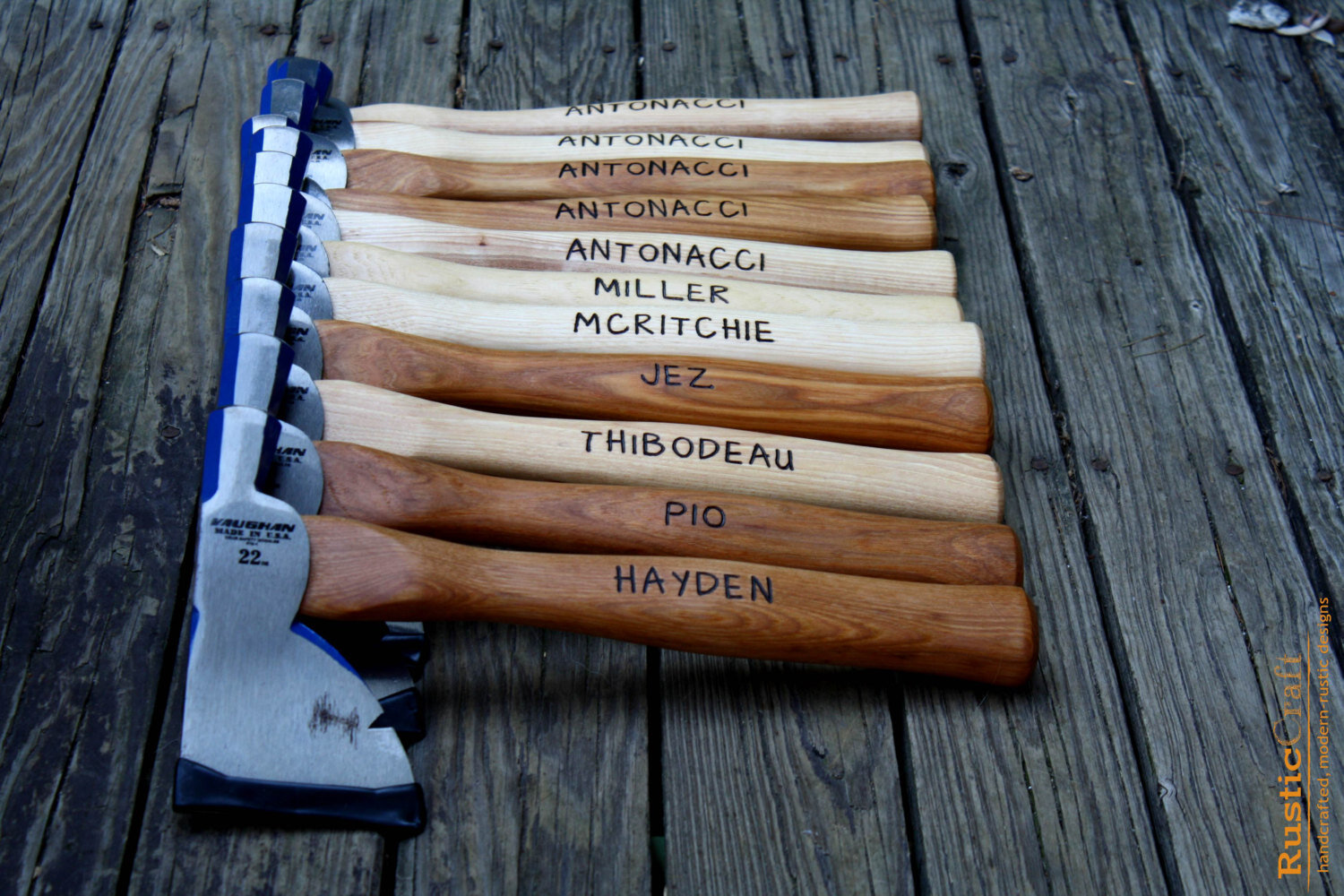The image depicts a neatly arranged lineup of eleven axes on a rustic wooden floor with weathered planks. Each ax boasts a wooden handle, varying in shades from light to dark, and each handle is engraved with a distinct name except for five, which all share the name Antonacci. The names inscribed on the handles in black lettering include Antonacci, Miller, McCritchie, Jez, Thibodeau (spelled T-H-I-B-O-D-E-A-U in one description), Pio, and Hayden. The silver metal heads of the axes feature blue accents at the top and are marked with the number 22 along with some other indistinct text. The overall setting suggests an older, rustic atmosphere, enhancing the visual appeal of the collection.